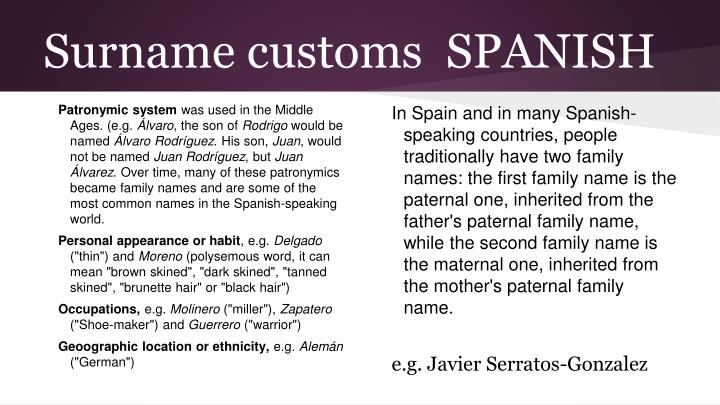The image is a PowerPoint slide predominantly featuring text, organized for educational purposes with a title on a dark purple banner at the top. The title is in white Georgia font and reads "Surname Customs Spanish," with "SPANISH" in all capital letters. Below the title, the content is divided into two columns of black text on a white background.

The left column starts with bold text, explaining that the patronymic system was used in the Middle Ages. For example, Alvaro, the son of Rodrigo, would be named Alvaro Rodriguez. His son Juan would not be named Juan Rodriguez, but Juan Alvarez. Over time, many patronymics became family names, now among the most common in the Spanish-speaking world. Further subheadings in bold include "Personal appearance or habit," "Occupations," and "Geographic location or ethnicity," detailing various naming conventions.

The right column explains that in Spain and many Spanish-speaking countries, people traditionally have two family names. The first family name is paternal, inherited from the father's family, while the second is maternal, inherited from the mother's paternal family. An example provided is Javier Serrano Gonzalez.

The text is centrally aligned on the slide, indicating a clear and structured format suitable for presentations or textbooks. The colors purple, white, and black are the primary visual elements, enhancing readability and emphasis on the important points.